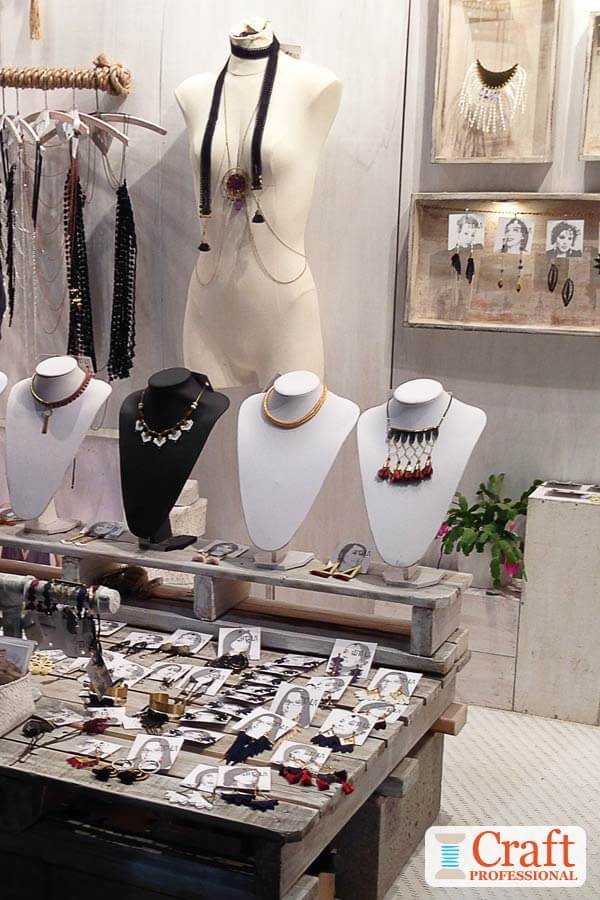This is a vertically-oriented, close-up color photograph capturing a detailed display inside a craft jewelry store, with a "Craft Professional" logo featuring red letters on a white background and a green thread spool in the bottom right corner. The main focus is a wooden table filled with a well-organized arrangement of jewelry. On the table, four neck mannequins showcase various necklaces, complementing a larger full-body mannequin in the background adorned with a scarf-like accessory and a prominent pendant. Additionally, the table features many pairs of earrings on little square packages and a cylinder stand displaying numerous bracelets. Behind this setup, various shelves made from wooden planks and concrete blocks exhibit numerous photographs of a light-skinned woman with black hair and glasses, each advertising different pairs of earrings. These shelves further present additional necklaces and jewelry items. In the top left center of the image, a rope with hangers displays long necklaces, while the top right corner includes boxes and a green plant with pink flowers, adding a touch of vibrancy to the scene.